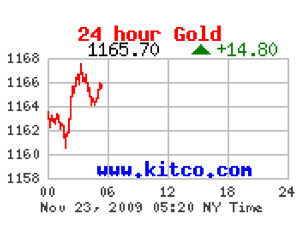The image is a detailed line chart tracking the price of gold. The title at the top is displayed in red text, reading "24-Hour Gold." The vertical axis on the left side features values ranging from 1158 to 1168, in increments of two. The horizontal axis at the bottom consists of time periods within a 24-hour span, marked as 00, 06, 12, 18, and 24. Beneath this axis, the date is specified in black text: "November 23rd, 2009 05:20 NY time." 

The chart also includes a data point with the value "1165.70" highlighted alongside a green arrow indicating an increase of 14.80 points. Text at the bottom of the image indicates the source website, "www.kitco.com," in blue font. The data line on the chart starts around 1164, dips to approximately 1161, peaks near 1168, and fluctuates in this manner. The image has a very basic and blocky font reminiscent of older computer graphics, making it appear outdated despite the 2009 timestamp.